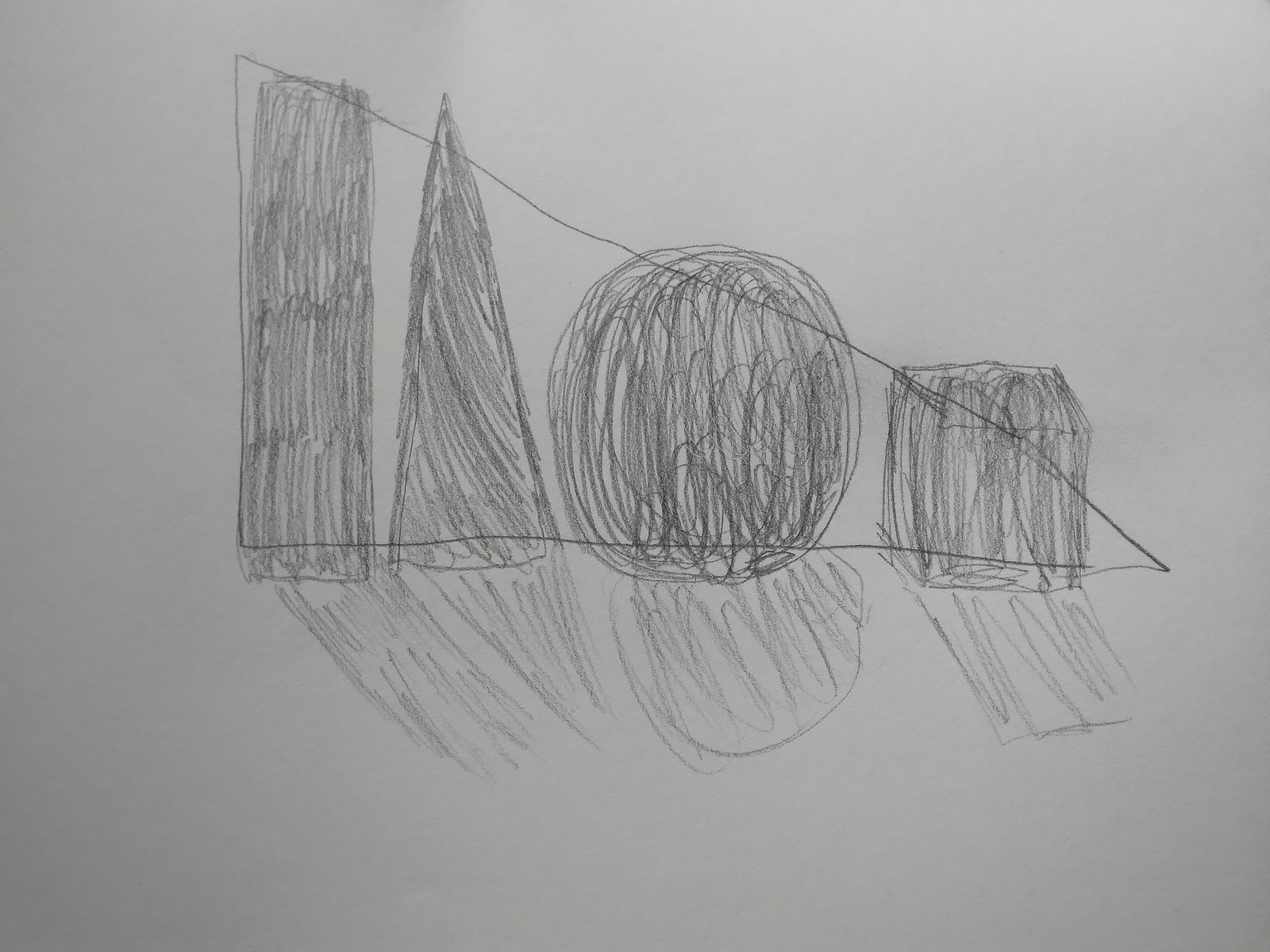This image features a pencil sketch rendered on plain white paper using what appears to be a basic number two graphite pencil. Dominating the composition is a large triangle that extends from a higher point on the left, sloping downward as it moves to the right. Within this prominent triangle, there are four distinct shapes: a long, skinny rectangle, another triangle resembling the shape of the letter 'A', a circle, and a cube. 

Unlike the other shapes, which are drawn in a two-dimensional manner, the cube is depicted with a sense of three-dimensionality. The lines of the shapes appear somewhat scribbled and rough, suggesting that the drawing was executed quickly. However, the overall craftsmanship indicates that it was created by an older child or an adult, rather than a younger child, due to the relatively controlled nature of the lines.

Adding to the depth of the sketch, shadows have been drawn beneath each of the four shapes. These shadows are angled towards the right, and are rendered with lighter, fainter pencil strokes compared to the main outlines. This detail adds a subtle dimension to the otherwise straightforward sketch. The collection of shapes enclosed within the larger triangle creates a cohesive and deliberately arranged composition, albeit one that appears to have been crafted in a somewhat hurried manner.